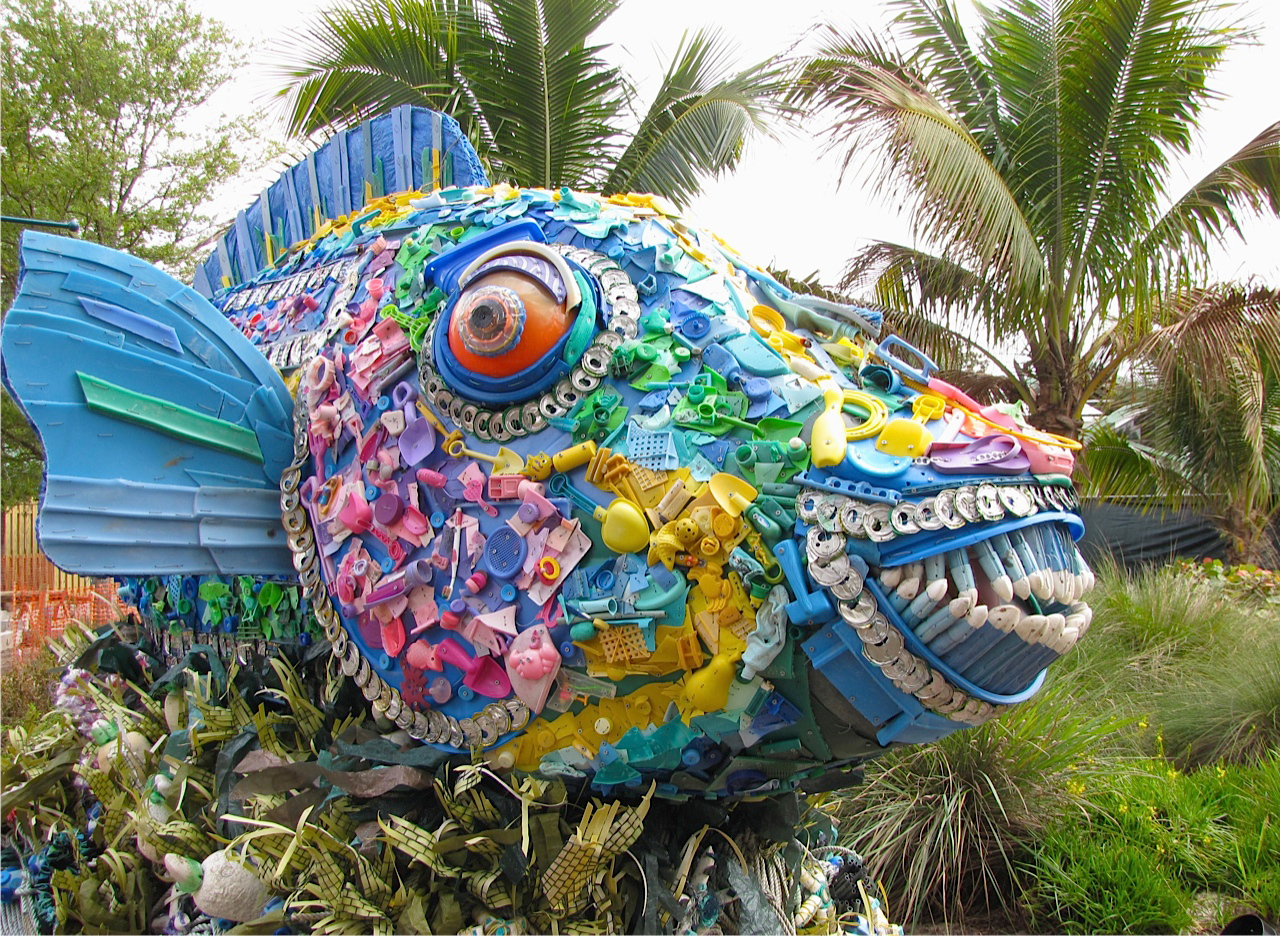The detailed image showcases a photorealistic sculpture of a large, blue fish situated outdoors in a tropical environment, with palm trees swaying in the background and tall grasses beneath the artwork. The fish is skillfully crafted from upcycled and scavenged plastic pieces, including items like sand shovels, cups, toys, flip-flops, and dishes, many of which seem to be remnants of beach litter. These plastic items are meticulously arranged to form the scales of the fish, adding a rich texture and vibrant colors—yellow, green, pink, purple, blue, and white—across its body. The fish features pronounced, scary-looking teeth colored in blue and white, as well as a striking red eye. Facing to the right of the frame, the sculpture allows visibility of the head, one pectoral fin, and a prominent dorsal fin, all adding to its intricate design. The artist has captured the essence of environmental awareness by transforming discarded materials into a stunning and evocative piece of art.